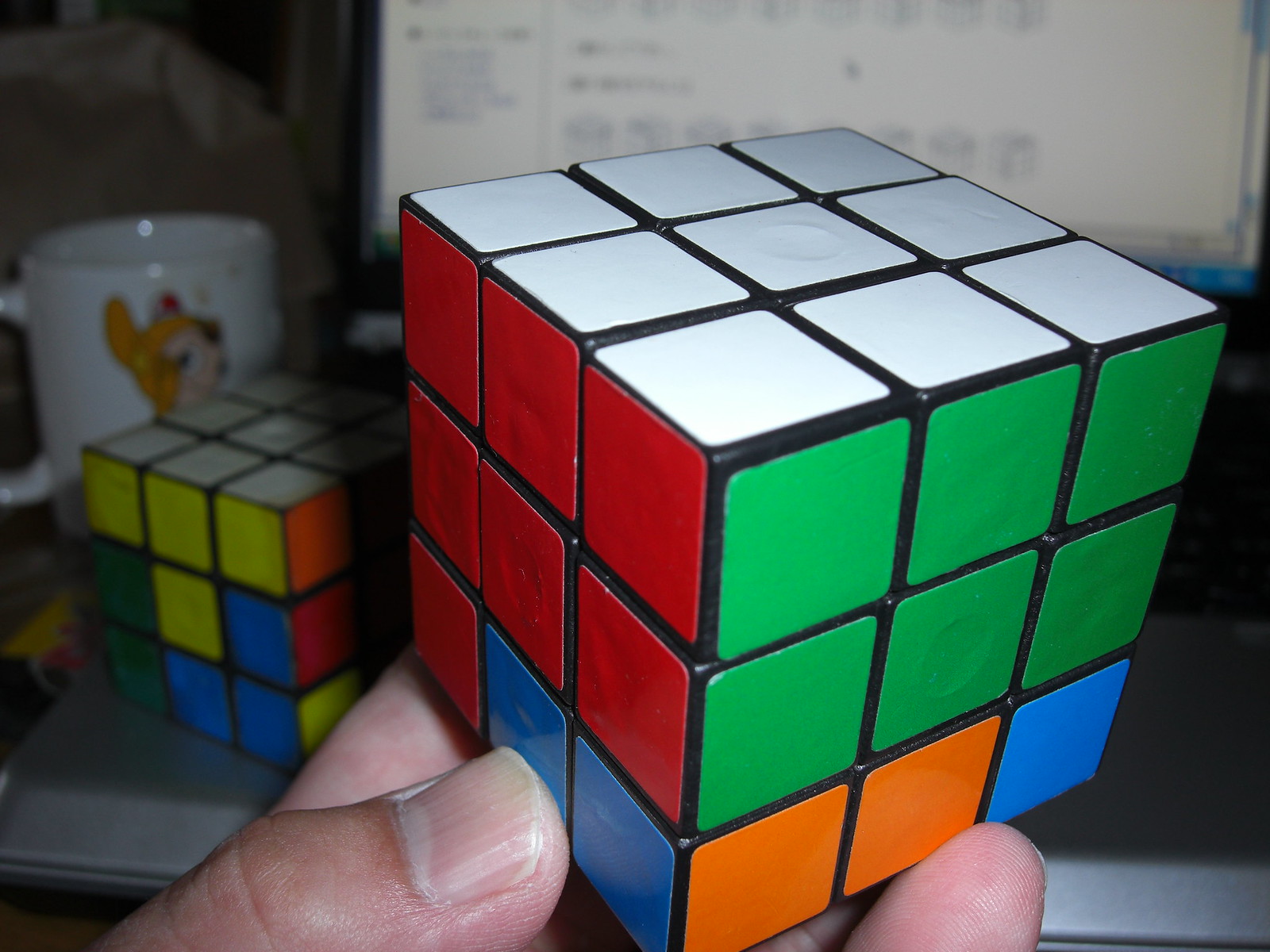In this detailed indoor image, a close-up shows a person's hand—evidently male, with the thumb, index finger, and pinky visible—holding a partially solved Rubik's Cube. The top face of the cube in the hand is completely white, while the left side is predominantly red with two blue tiles at the bottom. The right side displays two rows of six green tiles at the top, followed by two orange tiles and a single blue tile on the bottom row. 

In the background, slightly out of focus, sits another Rubik's Cube on the keyboard of a laptop. This secondary cube has one side solved—white—while other faces remain scrambled, featuring a yellow T-shape and a mix of green, blue, orange, red, and yellow tiles. Resting diagonally on the laptop, itself somewhat blurred, the screen behind this second cube appears to show a Rubik's Cube tutorial, hinting that the person may be using it for guidance.

To the laptop’s left, there is a white mug adorned with a cartoonish image that seems to depict a fleshy figure with an orange top, possibly resembling a dog wearing a Roman helmet. However, the blurred details make it difficult to discern clearly.

In the far background, a surface draped with a white cloth is faintly visible, enveloping the scene in a sense of casual indoor ambiance.